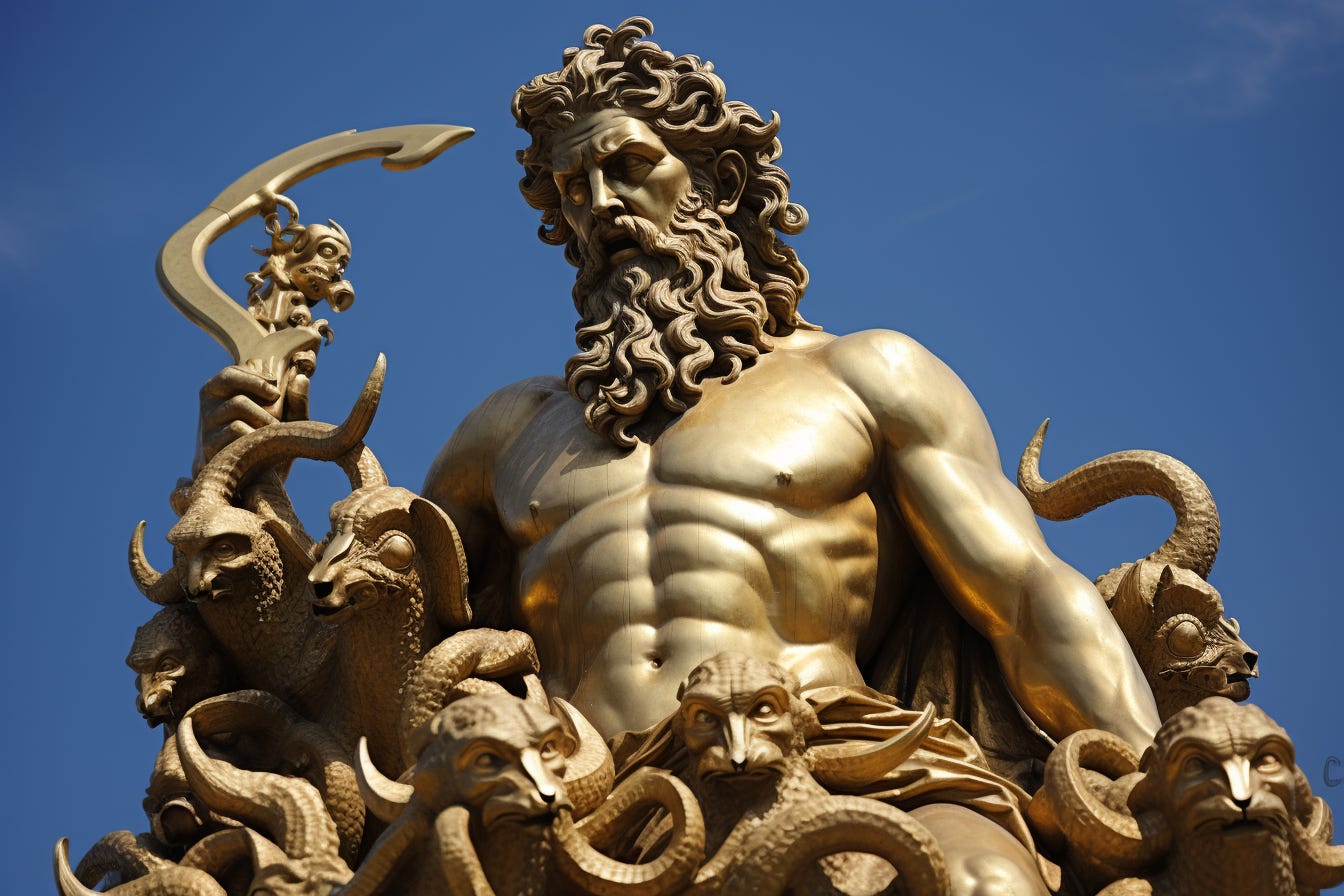In this image, we see a striking outdoor sculpture against a clear blue sky, with only a few wispy clouds in the upper right corner. The bronze-gold sculpture is of a muscular, shirtless man with a flowing mane of wavy hair and a long, curly beard and mustache. His solemn and intense gaze is directed down towards the bottom left. The man's right hand holds a hooked, spear-like object resembling a trident, while his left arm hangs at his side. Intriguing details surround him, including assorted goat-like creatures with curved horns that serve as decorative elements around his waist. Just a part of his upper thigh is visible on the bottom right of the image. The man’s detailed musculature, bare chest, and six-pack abs hint at the depiction of a powerful figure, possibly a Greek god like Zeus or Poseidon.